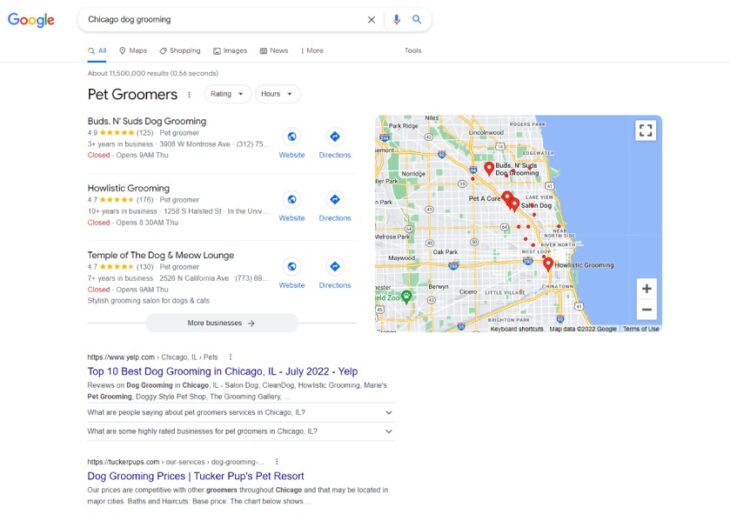**Detailed Caption:**

A Google search results page displaying information for "Chicago dog grooming" under the 'All' tab. The page indicates a total of about 11,500,000 results retrieved in 0.56 seconds. The image quality is poor, but details of the top search results are visible.

1. **First Result:**
   - **Business Name:** Buds & Suds Groomers
   - **Rating:** 4.9 stars based on 125 reviews
   - **Category:** Pet Groomer
   - **Years in Business:** Over 3 years
   - **Address:** 3904 West Montrose Avenue
   - **Operating Hours:** Currently closed, opens at 9 a.m. on Thursday

2. **Second Result:**
   - **Business Name:** Howl Listed Grooming
   - **Rating:** 4.7 stars based on 176 reviews
   - **Category:** Pet Groomer
   - **Years in Business:** Over 10 years
   - **Address:** 1258 South [unclear section] Street
   - **Operating Hours:** Currently closed, opens at 8:30 a.m. on Thursday

3. **Third Result:**
   - **Business Name:** Temple of the Dog and Meow Lounge
   - **Rating:** 4.7 stars based on 130 reviews

Additionally, the page features a map with the listed businesses pinned in red.